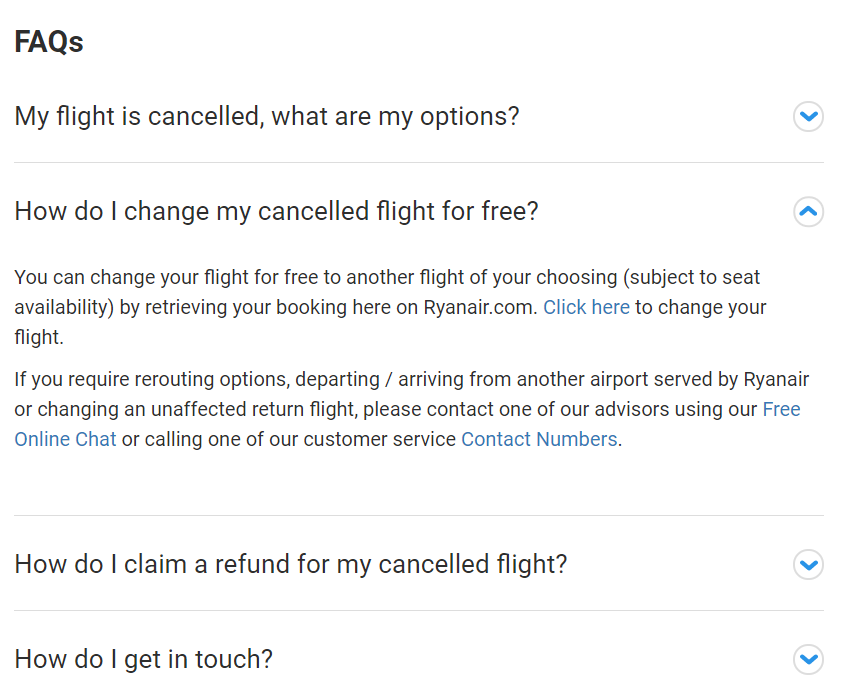This image is a cropped screenshot from the 'Facts' section of an airline's website. At the top left corner, the word "FACTS" is prominently displayed in bold black letters. Directly below that, in a slightly lighter black font, is the query "My flight is cancelled, what are my options?" accompanied by a blue downward-pointing arrow indicating a drop-down menu for additional information.

Continuing down the list, the next question reads "How do I change my cancelled flight for free?" To the right of this question is an expanded drop-down box containing the answer, which states: "You can change your flight for free to another flight of your choosing, subject to seat availability, by retrieving your booking here on Ryanair.com. Click here to change your flight," with "Click here" being a light blue hyperlink for easy access.

Further down, the query "How do I claim a refund for my cancelled flight?" appears with a minimized drop-down box to the right, indicating more information can be revealed. The final option at the bottom left of the screenshot poses the question "How do I get in touch?" This question also has a drop-down box to the right, which is currently not expanded.